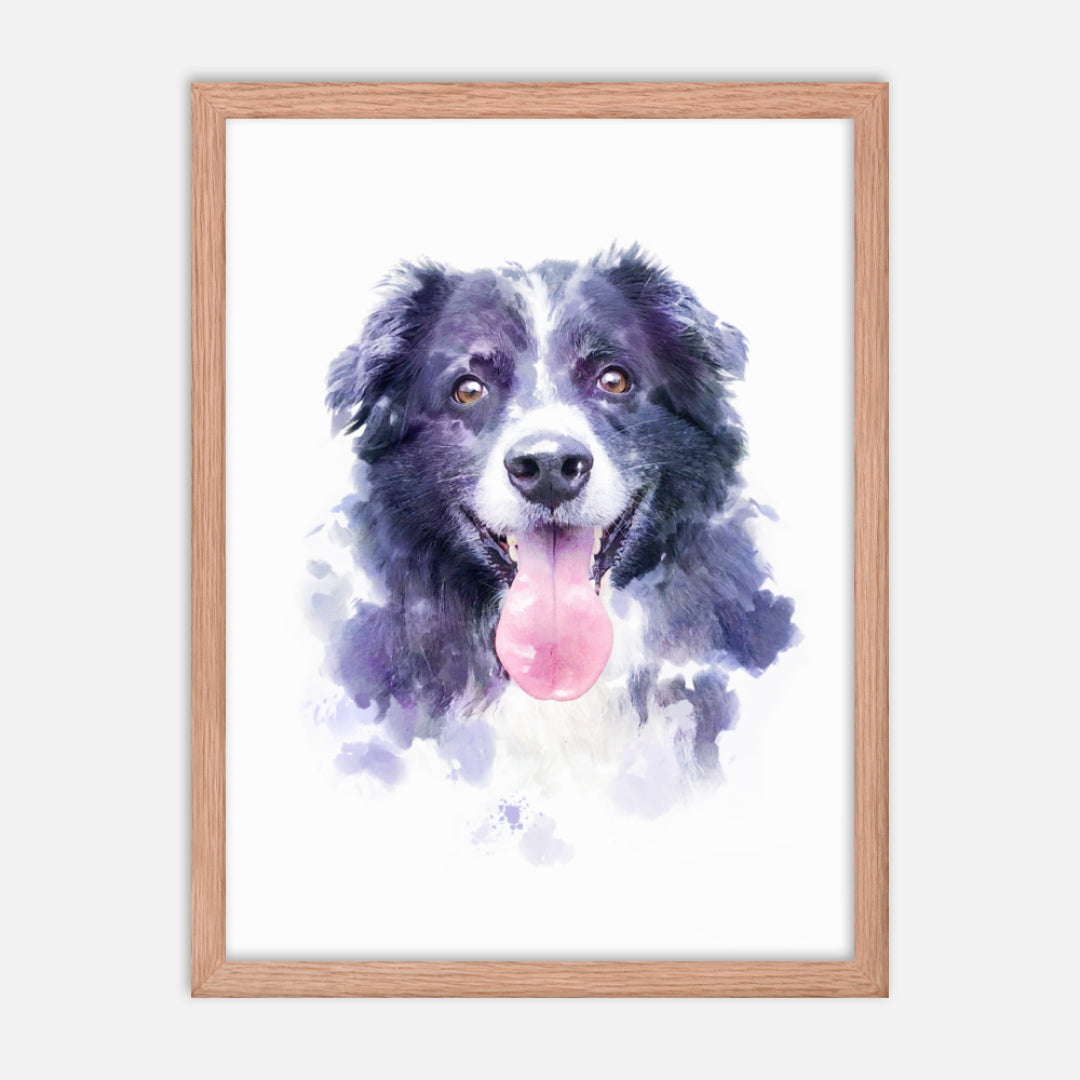The framed picture is a detailed painting of a cheerful Border Collie, characterized by its distinctive markings and relaxed demeanor. The dog, facing forward and appearing to look at the viewer, is depicted with a black coat, a white stripe down the middle of its face, and white fur around its muzzle and extending between its eyes. It has expressive brown eyes and a long, bright pink tongue hanging out of its open mouth, highlighting its happy expression. The dog's ears are floppy, laying flat against its head with white fur at their edges.

The painting employs a light, slightly hazy style reminiscent of watercolor, especially around the edges and lower portion, where the neck and shoulders fade into the white background. The background itself is pure white, making the dog the clear focal point. The absence of an artist's signature suggests an air of mystery, leaving the viewer to focus solely on the dog's lively depiction.

The artwork is housed within a simple, light blonde wooden frame that fully complements the picture's gentle aesthetic. The frame surrounds a yellow mat that contrasts subtly with the white canvas, while the entire piece hangs on an equally white wall, showcasing the dog's vivacious character against a minimalist backdrop.